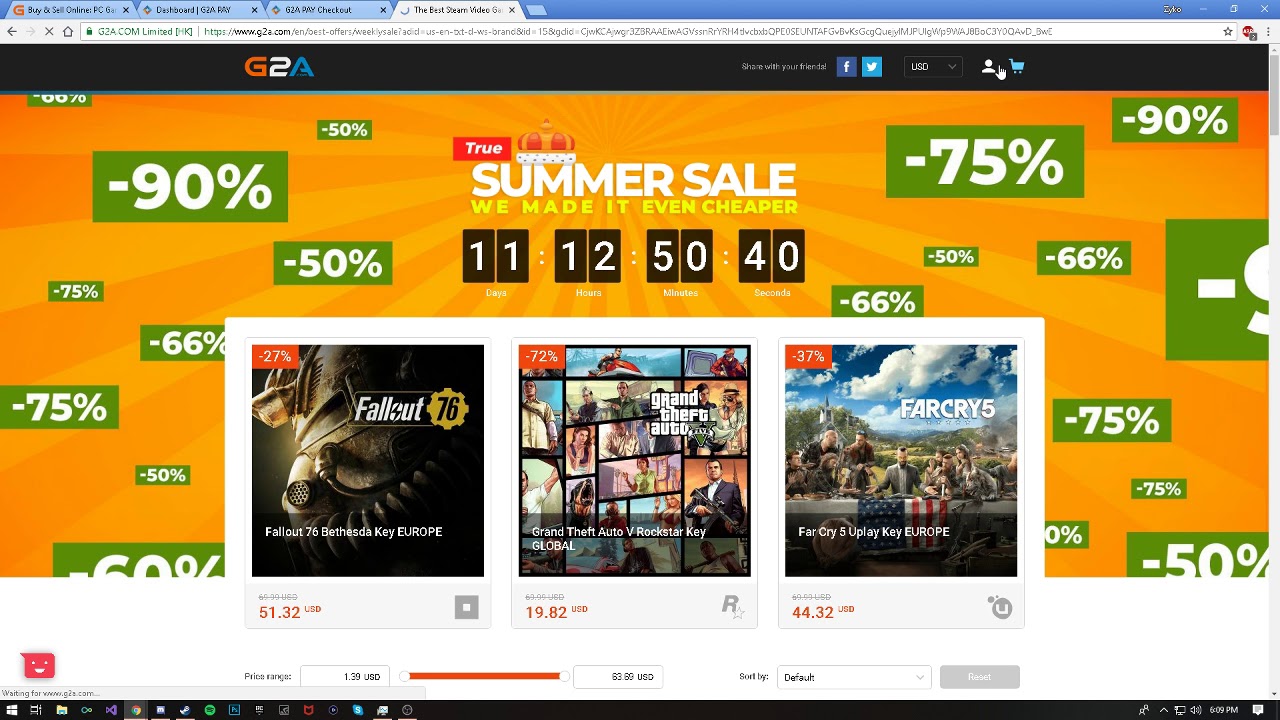The image showcases a vibrant summer sale advertisement on a computer screen, with an eye-catching orange background. Dominated by an array of discount offers, the screen displays various green rectangular banners highlighting dramatic price cuts, such as 90% off and 50% off. Prominently, the advertisement emphasizes "We made it even cheaper" and indicates the countdown for the sale, suggesting 11 days, and included hours, minutes, and seconds left until the sale begins or ends.

The screenshot is from the G2A website, which specializes in selling video games and related content. Featured prominently are popular games with significant discounts: Fallout 76 at 20% off, Grand Theft Auto V slashed by 72%, and Far Cry 5 reduced by 37%. These enticing deals are scattered across the webpage, inviting potential buyers to take advantage of the summer sale extravaganza.